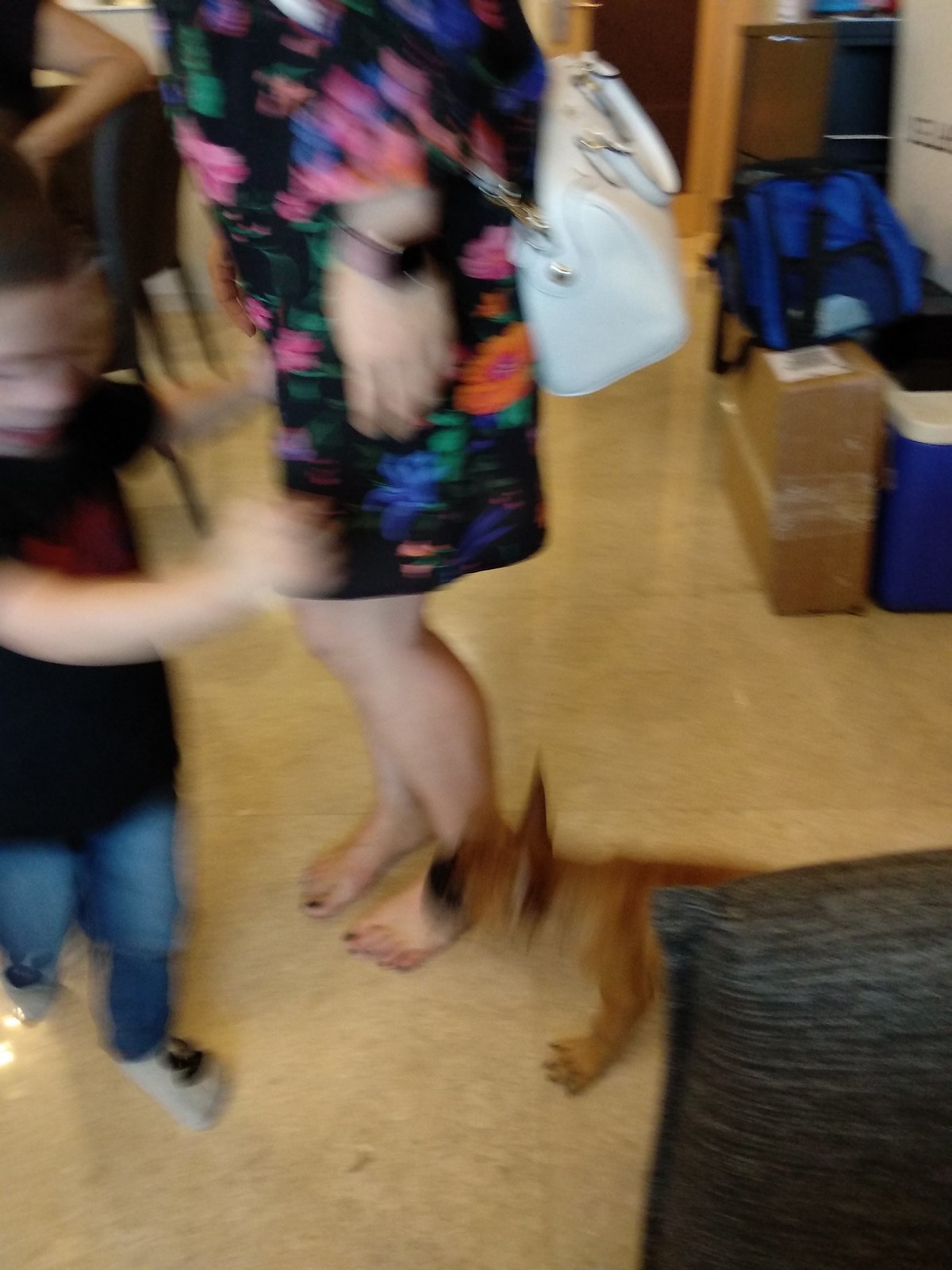In a somewhat blurry photograph that evokes the sensation of movement, a room with a beige, laminate tile floor serves as the backdrop. A woman, partially seen from her chest down, stands barefoot in the middle of the frame. Her toes are painted black, and she dons a knee-length, long-sleeve, black floral dress adorned with vibrant blue, orange, pink, and red flowers. She carries a white purse and an Apple Watch graces her left wrist. Nearby, a young boy, estimated to be around four years old, is caught mid-motion, clad in blue jeans, a black short-sleeved shirt with red writing, and socks. His hands are flailing as he looks down at what appears to be a small brown dog, likely a French bulldog with a tan coat, a black snout, and pointy ears, even though it’s quite blurry. A gray pillow in the bottom right corner partially obscures the dog. The background reveals a clutter with a mix of boxes, luggage, and what could be a blue dog carrying bag. To the upper right, an arm of another individual in a black top is visible, possibly folded. The scene is set off by hints of additional furniture, including what seems to be a gray chair or some other seating.